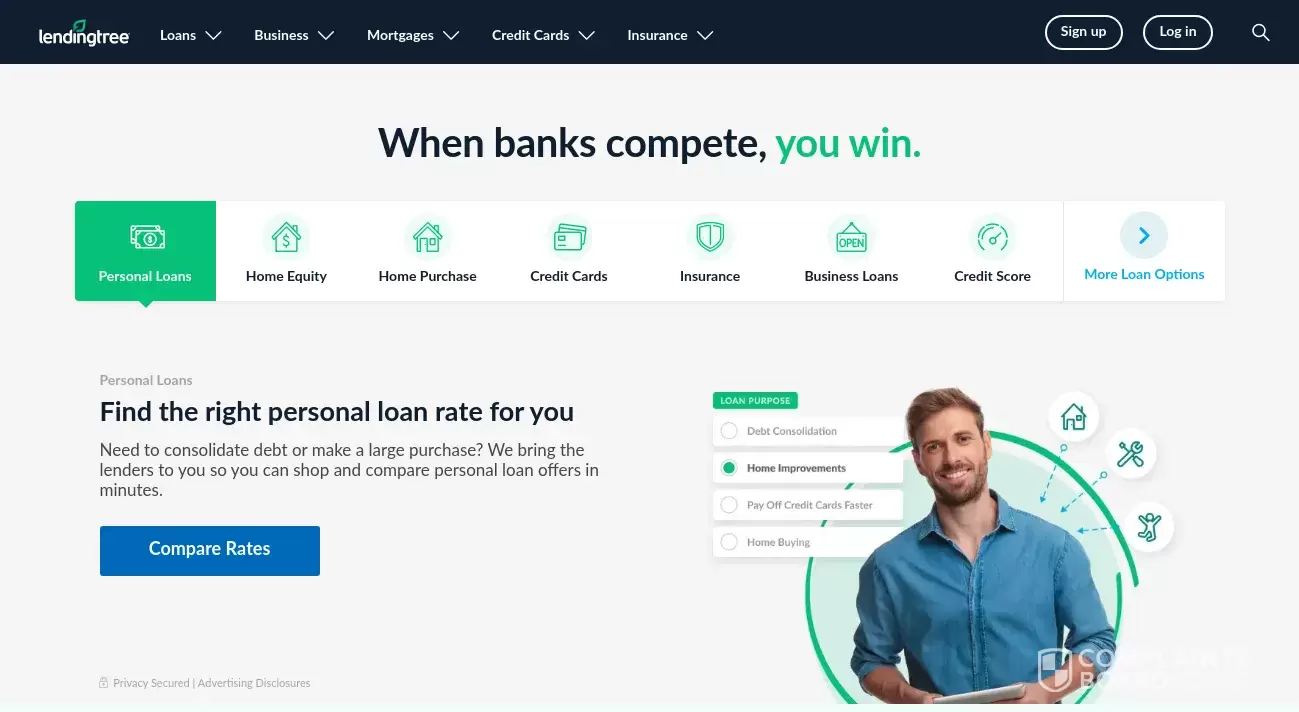This image showcases a screenshot from the LendingTree app or website, featuring a clear, organized layout. The interface is set against a white background, with a prominent black bar at the top displaying the LendingTree logo in white text. This bar also includes several clickable headings, such as Loans, Mortgages, Credit Cards, Auto, Financial Help, along with a Sign Up or Log In option, each with a downward arrow indicating further menus.

Beneath this, a bold statement reads: "We Show Your Options, You Score the Win," with the word "Win" highlighted in green to emphasize success. On the upper left, a horizontal bar with tabs provides navigation, with the tab for Personal Loans highlighted in green. This selection leads to a section titled, "Find the Right Personal Loan Rate for You," featuring a prominent blue "Compare Rates" button for user convenience.

To the middle right, there's a welcoming image of an agent—a young man with a beard and mustache, sporting short brown hair and a friendly smile. He is dressed in a blue work shirt and positioned within a green circle against a blue background, embodying a helpful guide for Debt Consolidation and Home Improvements options.

Moreover, the bottom left corner of the screen displays images of a phone and a tablet, indicating the platform's accessibility across multiple devices. The overall image captures the intuitive design and user-friendly features of the LendingTree platform, aimed at helping users make informed financial decisions.